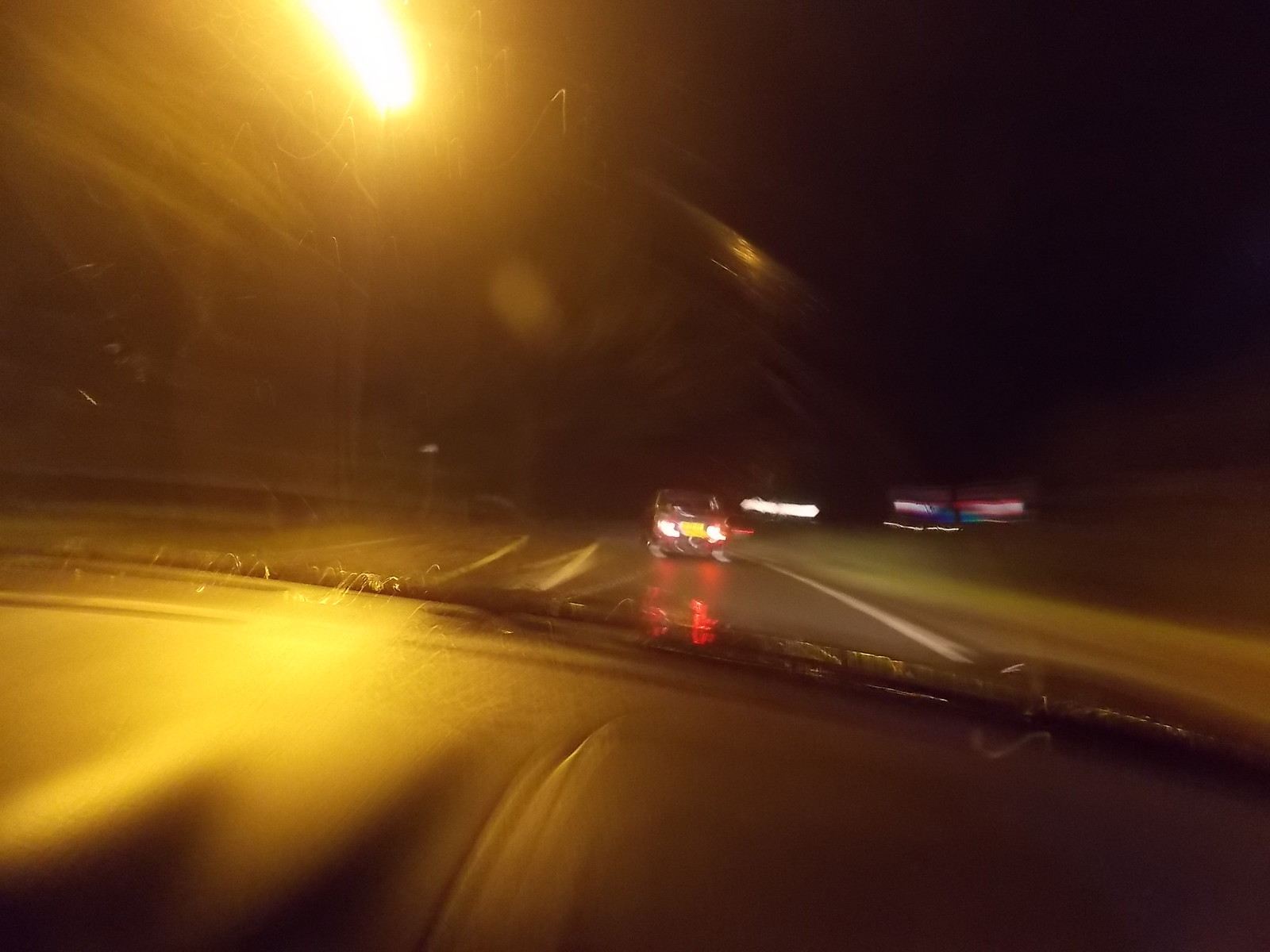This photograph, taken at night, appears from the backseat of a vehicle, possibly facing slightly forward and capturing the dashboard. The image is blurry but reveals several details: a road stretches ahead of the vehicle, with another car approximately 15 meters in front, its motion suggesting the vehicle is moving quickly. The scene is mostly dark, save for a yellow street light positioned in the upper left corner of the image. The bright lights from a car behind illuminate the rear, along with the faint outline of highway lines and tail lights from vehicles on the opposite side of the road. The silhouette of a leather backseat is also visible, emphasizing the interior setting of the car.